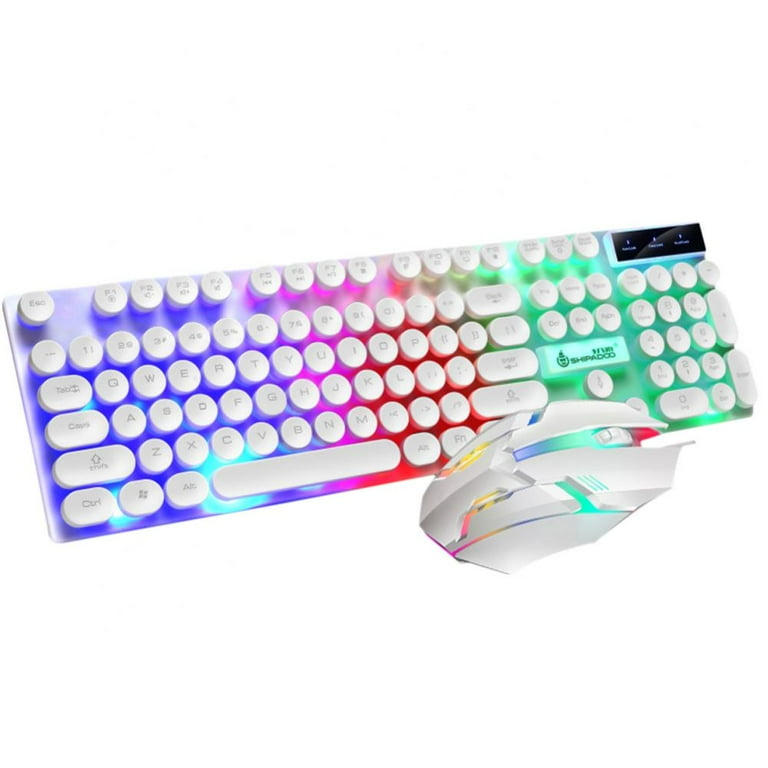This digital image showcases a wireless keyboard and mouse, both featuring a colorful and vibrant design. The keyboard keys are all white and predominantly rounded, except for the caps lock and shift keys, which have a more horizontal, oval shape. Illuminated neon and bright colors fill the space between the keys, creating a visually striking backdrop. Starting from the left, the colors transition from royal blue and dark blue to lighter shades of blue and fuchsia, then to red, and finally to green towards the right side, where the number keys are located. Smaller sections of pink and yellow are also interspersed throughout. Below the keyboard, there's a sleek, white wireless mouse with a similar color scheme, including patches of pinks, yellows, blues, greens, and reds. The mouse has noticeable cutouts, giving it a segmented appearance, and it is propped up in front of the keyboard. Both devices are positioned at a slight angle, enhancing their dynamic presentation.